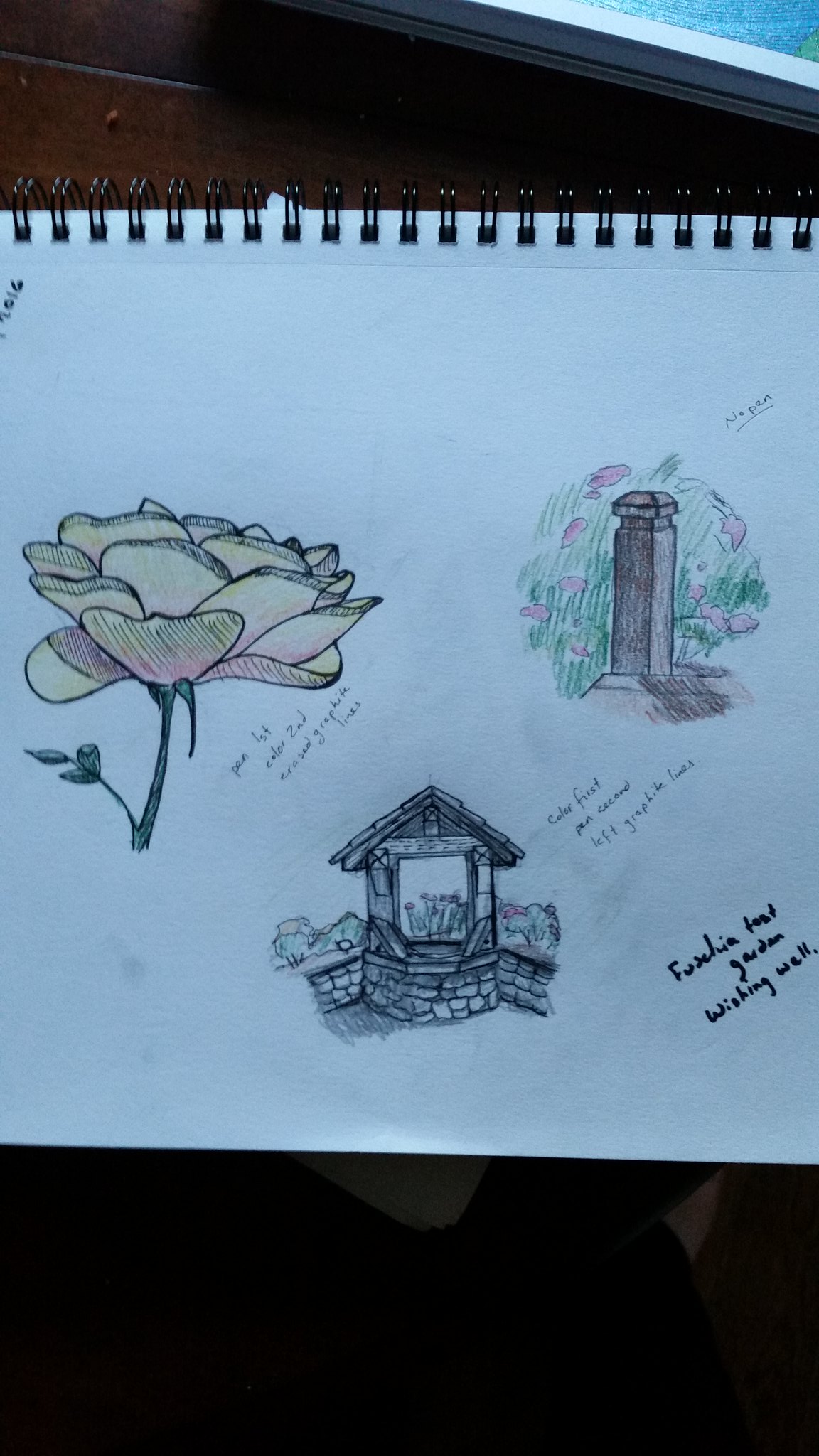The image depicts a tall, narrow photograph focusing on a sketch pad centered on a dark-stained wooden table with lateral boards, partially obscured in the lower portion. The background frames a window in the upper right corner, outside of which sunlight filters through, hinting at an outdoor setting. The sketch pad, bound at the top with black rings, occupies about two-thirds of the image. On the left side of the pad, a colored pencil drawing showcases a yellow and pink flower with a green stem and leaves. Below this, toward the bottom center, there's a detailed sketch of a black and white well with a small roof. In the upper right section of the pad, a brown monument or pillar stands amidst green grass and pink flowers, drawn in a circular pattern. Some indecipherable black lettering, possibly done with a Sharpie, appears in the bottom right of the pad.